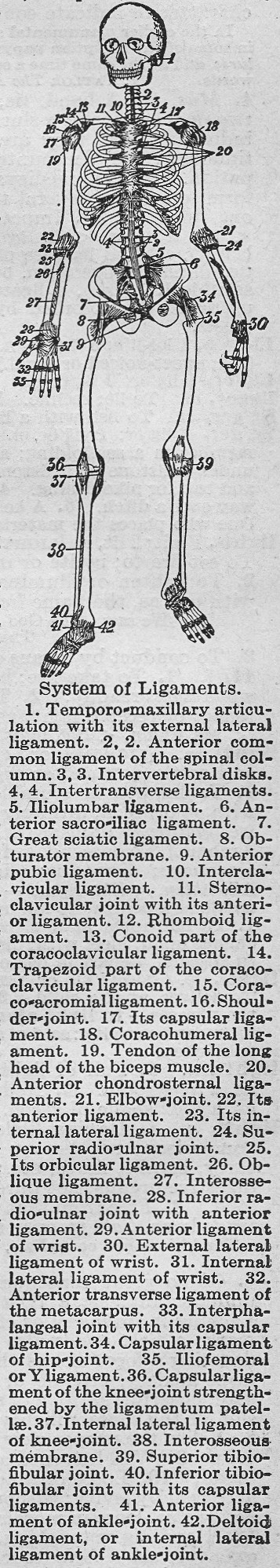The image depicts a detailed diagram of a full-body skeleton at the top of a passage titled "System of Ligaments." The skeleton is annotated with numbers, starting from the head at number 1 and continuing down to the feet, ending at number 42. These numbers correspond to specific bones and their ligaments, with number 1 indicating the temporomaxillary articulation at the head. The background is white and the text is printed in black, aligning each numbered part of the skeleton with its respective description in the passage below. The layout and style resemble that of a newspaper or an old printed document, giving the background a slight grayish tone and rendering the text small and somewhat difficult to read.